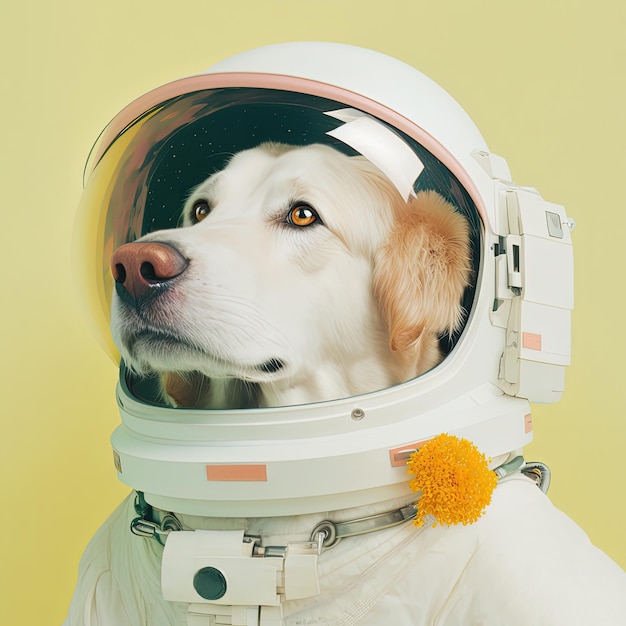The image appears to be a digitally created artwork featuring a golden retriever or Labrador dog in a white astronaut suit. The dog's face, characterized by its golden eyes, large brown nose, and whitish-brown fur, is clearly visible through a glass or plexiglass helmet. This clear helmet includes detailed reflections, such as a faint fluorescent light, and presents a star field backdrop inside it, contrasting with the pale yellow, painted background of the overall image. Distinctive features such as an orange or yellow pom-pom detail near the neck and peach-colored accents around the helmet add vibrant touches to the primarily white space suit. The overall appearance blends elements of digital photo enhancements with painting techniques, resulting in a striking, surreal portrayal of a spacefaring canine.